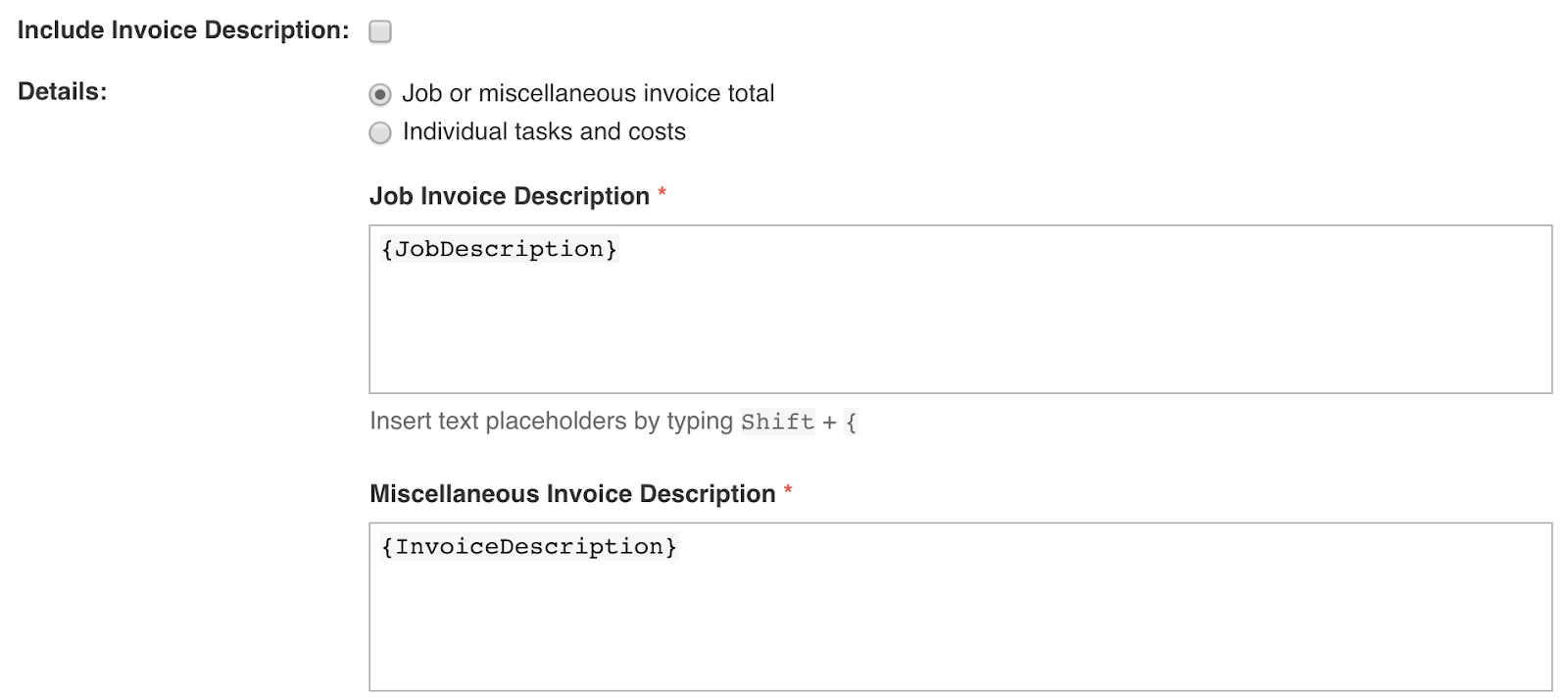This screenshot captures a section of an unspecified website, presenting a form designed for managing invoice descriptions. The background of the webpage is plain white with no borders, and the interface is devoid of a left-side menu. 

At the top, bold black text instructs users to "Include invoice description," accompanied by an unselected checkbox option. Below this, a section labeled "Details" offers two radio button choices: "Job or miscellaneous invoice total" (which is selected) and "Individual tasks and costs" (which is unselected).

Further down, in bold black text marked with a red asterisk, the form prompts users for a "Job Invoice Description," followed by a text box containing placeholder text in brackets: [job description]. Directly beneath this, instructions in light gray text guide users to "Insert text placeholders by typing shift plus open bracket."

Following this, another bold black heading with a red asterisk requests a "Miscellaneous Invoice Description." A second text box appears below this heading, featuring placeholder text [invoice description] in brackets. Both text boxes are outlined with light gray borders, maintaining consistency with the rest of the form's design. The entire interface uses black and light gray fonts to match the minimalist aesthetic of the webpage.